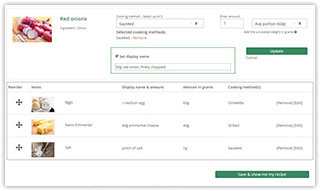This image is a detailed screenshot of a store's online advertisement. At the top, it prominently displays an image of red onions, some whole and some sliced. To the right of this image, there is a green square button labeled "Update." Below the onion image, there are smaller pictures of eggs, butter, and flour. Adjacent to them, another green square displays the text "Set Display." At the bottom right corner of the screenshot, a green button labeled "Submit" is visible. The entire layout has a white background with no additional images or text, and while the writing is small and somewhat difficult to read, the overall interface is clean and functional.